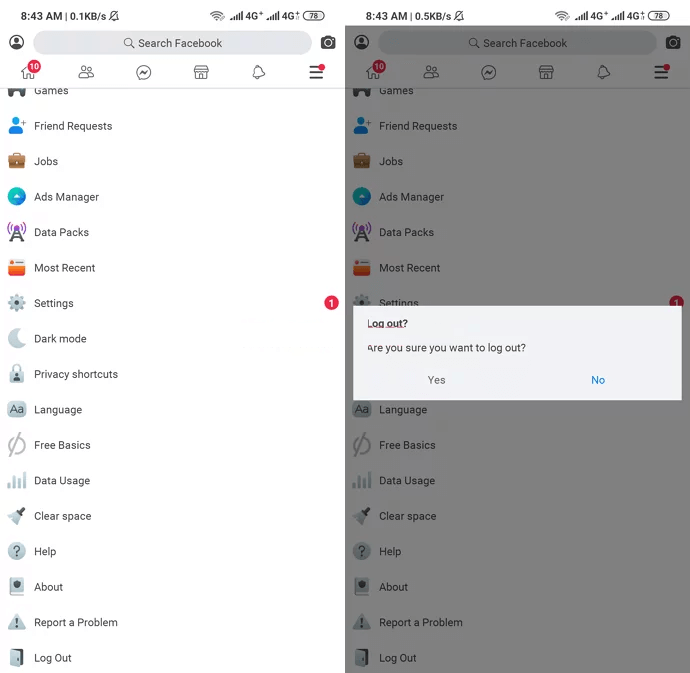This is a detailed screenshot of a Facebook mobile interface captured at 8:43 AM. The top section displays the time (8:43 AM) alongside a 4G connection icon with signal bars. A search bar labeled "Search Facebook" is prominently featured. To the right of the search bar, there are several icons: a home icon with 10 notifications, a notification bell, and the Messenger logo.

Scrolling further down, various menu options are visible. These include:
- **Games**
- **Friend Requests**
- **Jobs**
- **Ads Manager**
- **Data Packs**
- **Most Recent**

Further down, there are additional settings and options:
- **Settings**: Represented with a gear icon, which currently has one notification.
- **Dark Mode**: Indicated by a half-moon symbol.
- **Privacy Shortcuts**: Illustrated with a lock icon.
- **Language**
- **Free Basics**
- **Data Usage**
- **Clear Space**: Accompanied by a broom icon.
- **Help**: Represented by a question mark and includes a "Report a Problem" feature.
- **Log Out**